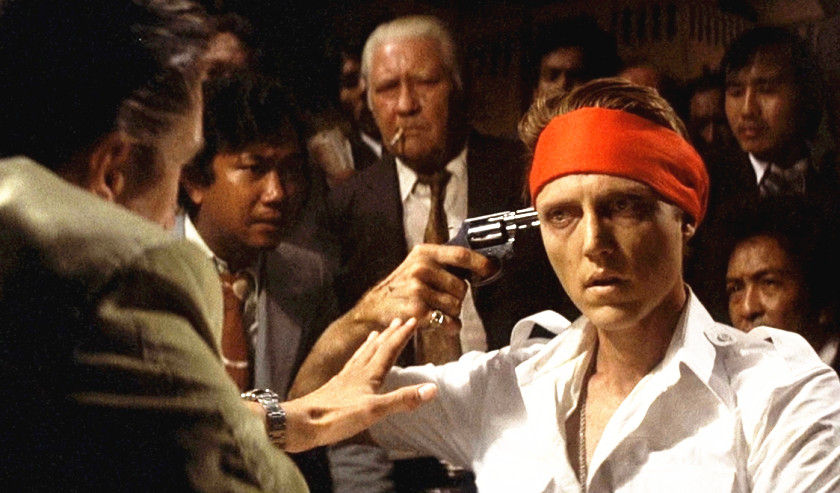The grainy, rectangular photograph appears to be a vintage movie still from the 1970s, featuring a tense scene with actor Christopher Walken in his younger years. Dominating the right half of the image, Walken is depicted from mid-chest upwards, wearing an open white collared shirt that reveals a silver chain and a pinky ring. His distinctive brown hair is held back by a large red bandana, emphasizing his serious facial expression as he holds a gun to his temple. Walken's right arm is extended out, elbow bent, gripping the weapon with a determined gaze fixed on a man standing to his left.

This man, whose face is partially obscured, is dressed in a light gray suit and has graying brown hair, signaling his older age. His left hand is extended out in a stopping gesture, palm facing Walken, perhaps pleading or commanding him to stop. Behind Walken, a group of apprehensive men of Asian descent look on, with one notable figure being an older, larger man with a cigarette hanging from his mouth. The otherwise serious expressions on all faces intensify the dramatic and despairing mood of the scene.